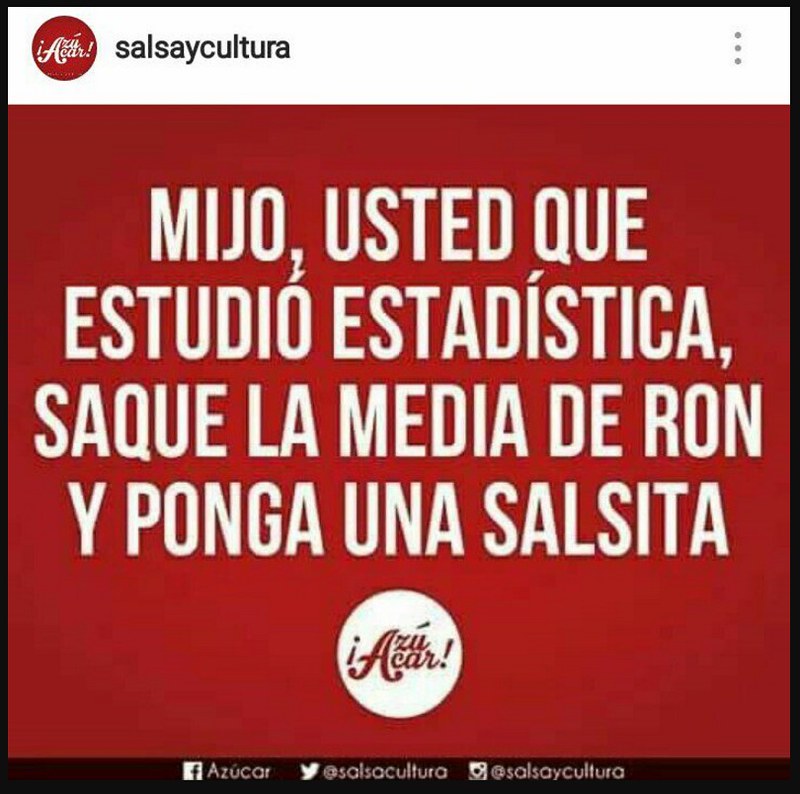The image appears to be an online advertisement, primarily in Spanish, with a red background and white text. In the upper left corner, there's a round logo with the word "¡Azúcar!" in white text inside a white circular banner. To the right of this logo, the black text reads "Salsa y Cultura," and on the far right, there are three vertical gray dots suggesting an options menu, mimicking a social media screenshot. Centered below, a large red box contains white capitalized text, "Mijo Usted Que Estudio Esta Testiquia Saque La Media De Ron Y Pongo Un Salsita." Another smaller white circle below this text features the word "¡Azúcar!" in red lettering. Along the bottom, a black banner displays social media logos: the Facebook "F" next to "¡Azúcar!" in white, the Twitter bird logo followed by "@SalsaCultura," and the Instagram camera icon followed by "@SalsaYCultura." The color scheme is primarily red, white, black, and gray, giving it a vibrant and eye-catching appearance typical of digital advertising.